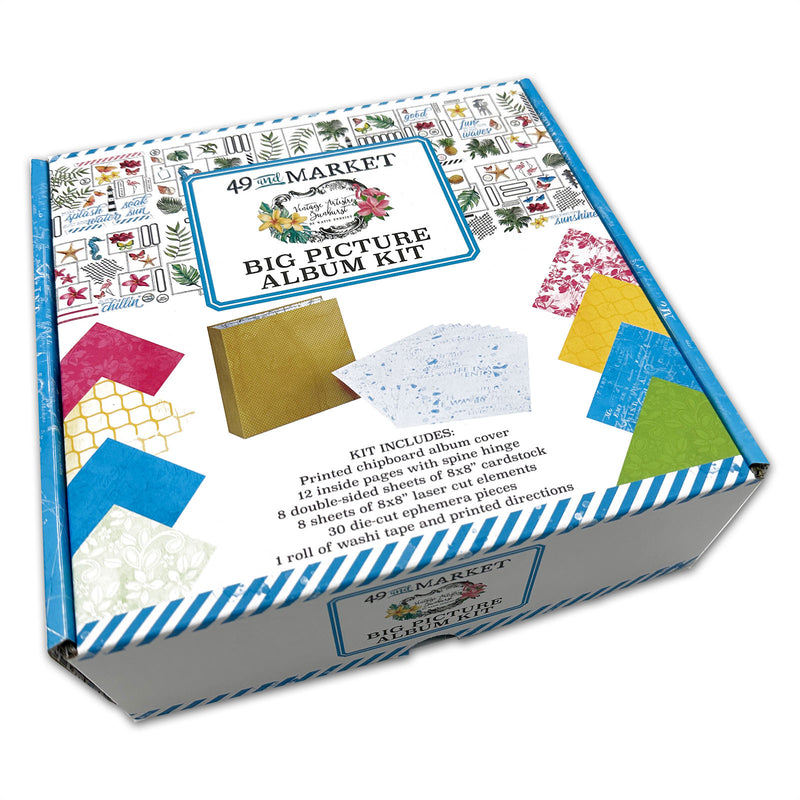This image showcases a vibrant, mailer-style package for a "Big Picture Album Kit" by 49 and Market. The top of the box is adorned with an array of colorful graphics, including seahorses, stars, and leaves, arranged in groups with festive holiday designs. Central to the design is a framed white box bordered in blue, housing the 49 and Market logo accompanied by a cursive script that is partially unreadable but accented by yellow and pink flowers.

The sides of the box feature various patterned papers in hues of red, gold, blue, and light green with white floral designs. A prominent picture of a gold photo album is displayed in the center, emphasizing the kit's contents. The box is labeled with detailed text that reads: "Kit includes: printed chipboard album cover, 12 inside pages with spine hinge, 8 double-sided sheets of 8x8 cardstock, 8 sheets of 8x8 laser-cut elements, 30 die-cut ephemera pieces, 1 roll of washi tape, and printed directions." The overall design and text make the package visually appealing and informative, highlighting the kit's rich assortment of crafting materials.